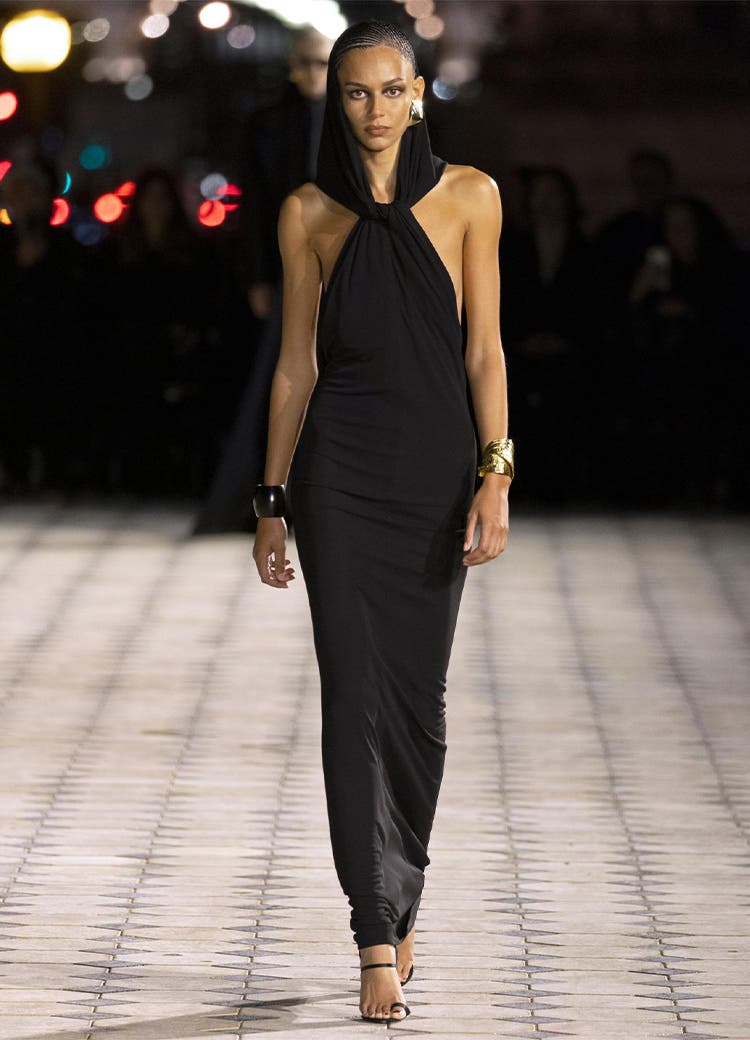The photograph features a tall, slender woman with darker skin, very short hair, and a distinct head covering. The headpiece, stemming from her halter-neck styled dress, extends up to partially cover her head, leaving her short hair exposed and one ear visible. She wears a form-fitting, one-piece black gown that reaches down to the top of her feet, fully covering her body, except for her side sections. Her demeanor is composed, with a blank expression and eyes staring directly at the viewer. Her accessories include a very large gold earring in her left ear, a gold bangle on her left wrist, and a chunky, black beaded bracelet on her right wrist. The woman is also donning black strappy heels. She walks on a cream-colored, stone-tiled surface with a grid pattern and diamond accents at the corners. The background is blurred, but it appears to be a runway show with spectators, one of whom is a man in dark glasses and attire, standing amidst a seated audience.